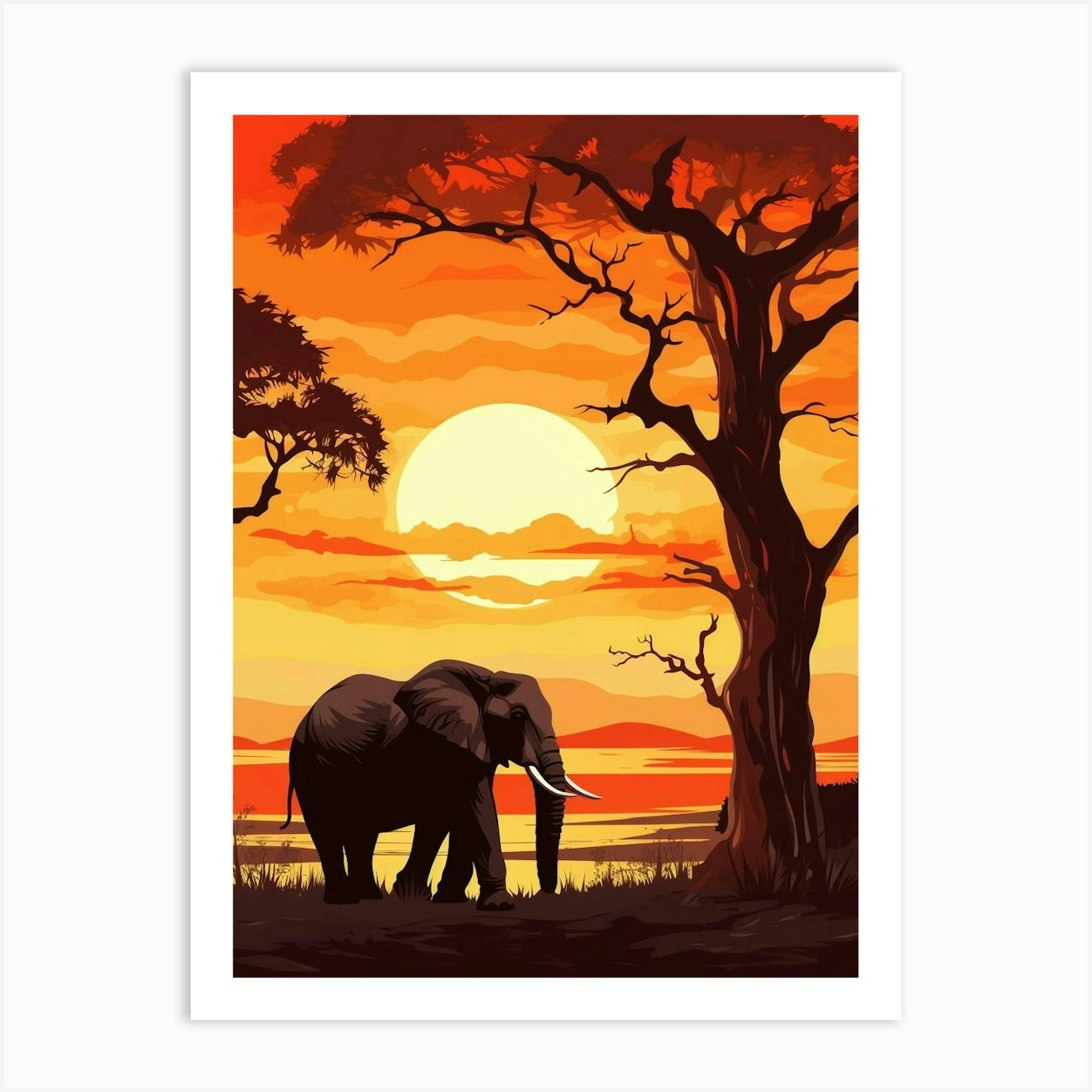This image is a detailed drawing of an African sunset scene, meticulously framed with a white border and mounted on a light-colored wall. Dominating the lower left-hand side of the artwork is a large gray elephant facing right, showcasing prominent white tusks. The ground beneath the elephant is a blend of brown hues with sparse vegetation. Spanning across the bottom, grassy terrain extends to the right side, where a towering tree rises. The tree, with thick branches, has its leaves clustered mainly at the top, silhouetted against a vibrant sky. The sky transitions from a deep orange at the top to a bright yellow lower down, where a round, white blazing sun occupies the center of the image. The backdrop features a layered horizon of dark orange and purple hills, adding depth to the scene. Additionally, on the middle left, another tree branch with leaves protrudes into the frame, its foliage stretching upwards before disappearing off the edge. This artwork beautifully captures a rich palette of browns, grays, oranges, yellows, and reds, vividly portraying an elephant in its natural habitat during an enchanting sunset.